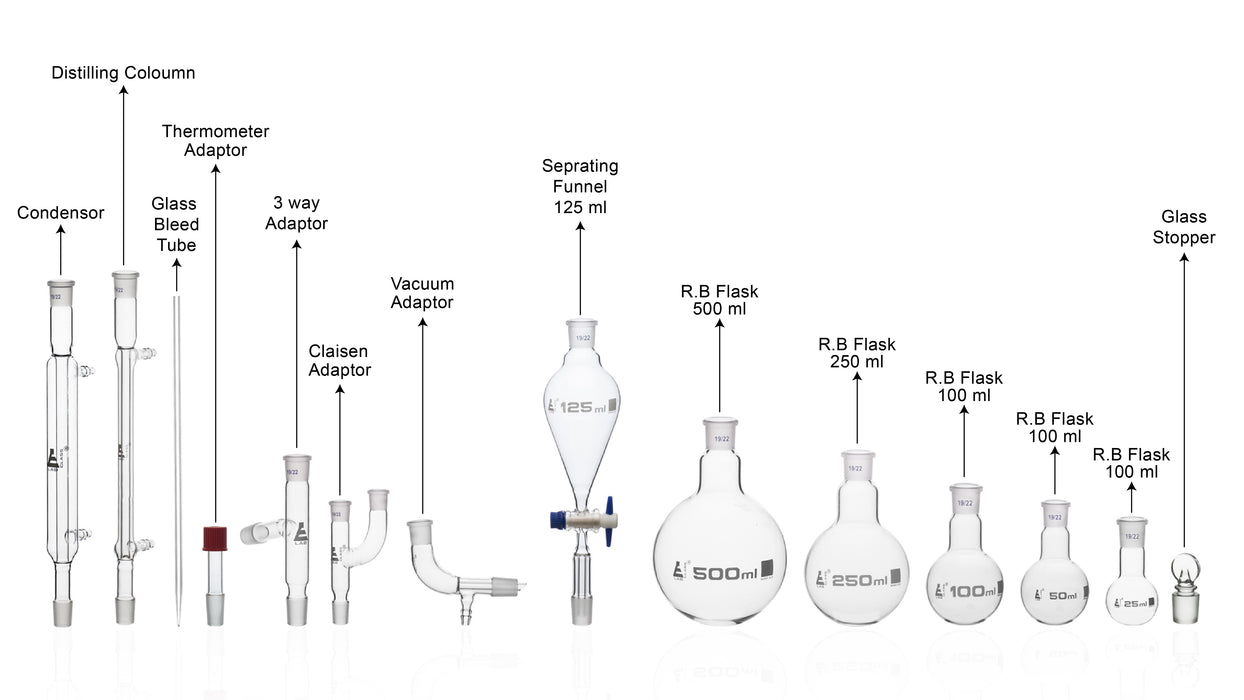The detailed diagram depicts an assortment of chemistry set equipment, arranged from left to right in sequential order. Starting with narrow glass tubes, it features a condenser—identified by its long tube with two fittings—followed by a distilling column that visually resembles the condenser. Next is a glass bleed tube, a slim and elongated piece, and a thermometer adapter, characterized by its short shaft designed to hold a thermometer. The set also includes a three-way adapter, distinguishable by its glass tube with a side split, and a Claisen adapter, which is a straight tube with an upward split. Further down, there's a vacuum adapter with a curved form and a bottom fitting. This is followed by a separating funnel, a 125-milliliter funnel-shaped glass with a valve for dividing chemicals.

The collection further features a series of round bottom (RB) flasks in several sizes and a few mislabeled ones: a 500-milliliter flask, a 250-milliliter flask, two 100-milliliter flasks, one flask originally labeled as 100 milliliters but is actually 50 milliliters, and the smallest mislabeled flask marked as 100 milliliters, which is in reality 25 milliliters. The final item in the lineup is a glass stopper, which fits snugly into the tops of the flasks for secure closure. All items in the diagram are crystal clear and meticulously labeled with their respective sizes, providing essential tools that might be used for distillation processes, possibly in activities like moonshine production or other distillery functions.